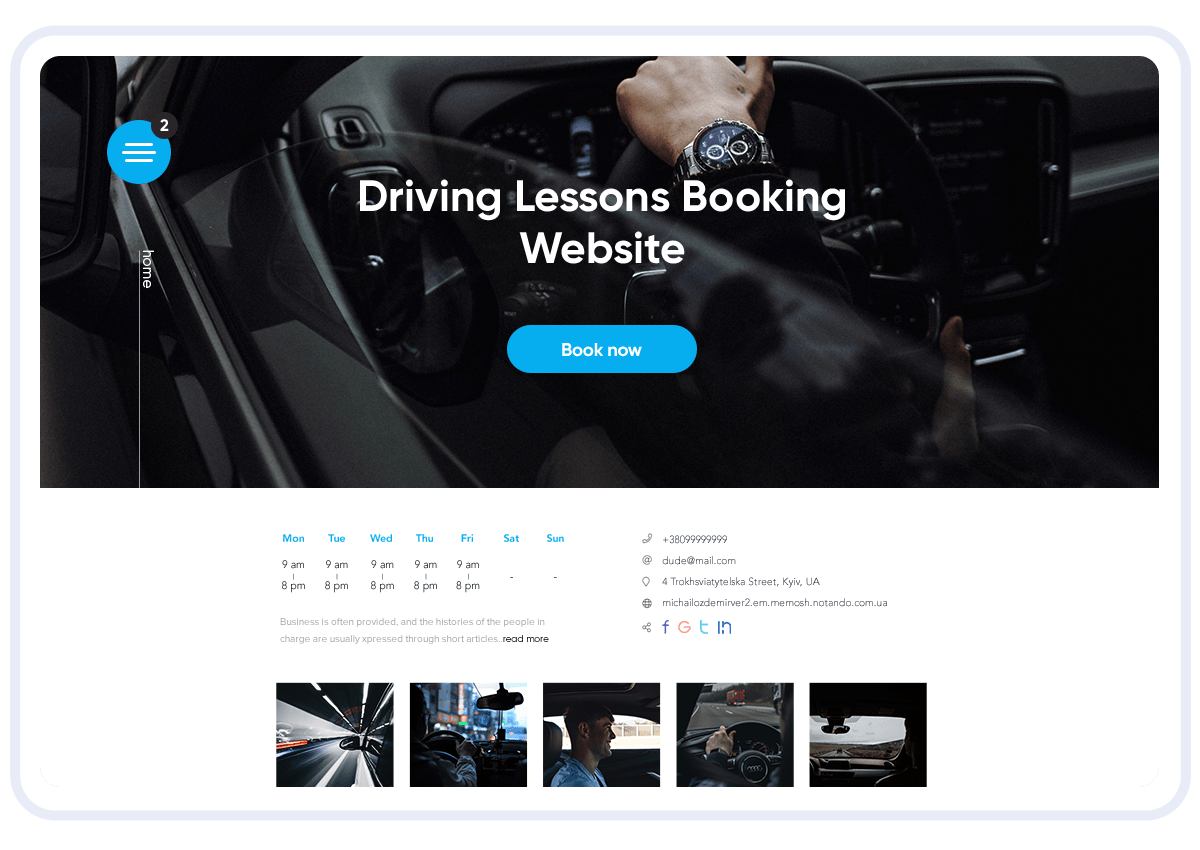This image is an advertisement for a driving lessons booking website, prominently displaying a sleek, black-interior car with a close-up of an arm wearing a fancy watch holding the steering wheel. The title "Driving Lessons Booking Website" appears in bold white text over the image. Below this, a blue "Book Now" button invites users to take action. Beneath the button, a weekly schedule indicates available booking times from Monday to Friday, 9 a.m. to 8 p.m., with hyphens suggesting the service is closed on weekends. The webpage also includes a menu icon with a number 2 in a black circle, and at the bottom, several smaller images depict various driving scenes, such as street views, hands on steering wheels, and profiles of drivers. Additional details include contact information such as an email (dude at mail.com), a phone number, a mailing address in Kiev, and a web address, along with brief articles highlighting the business history and profiles of key personnel.